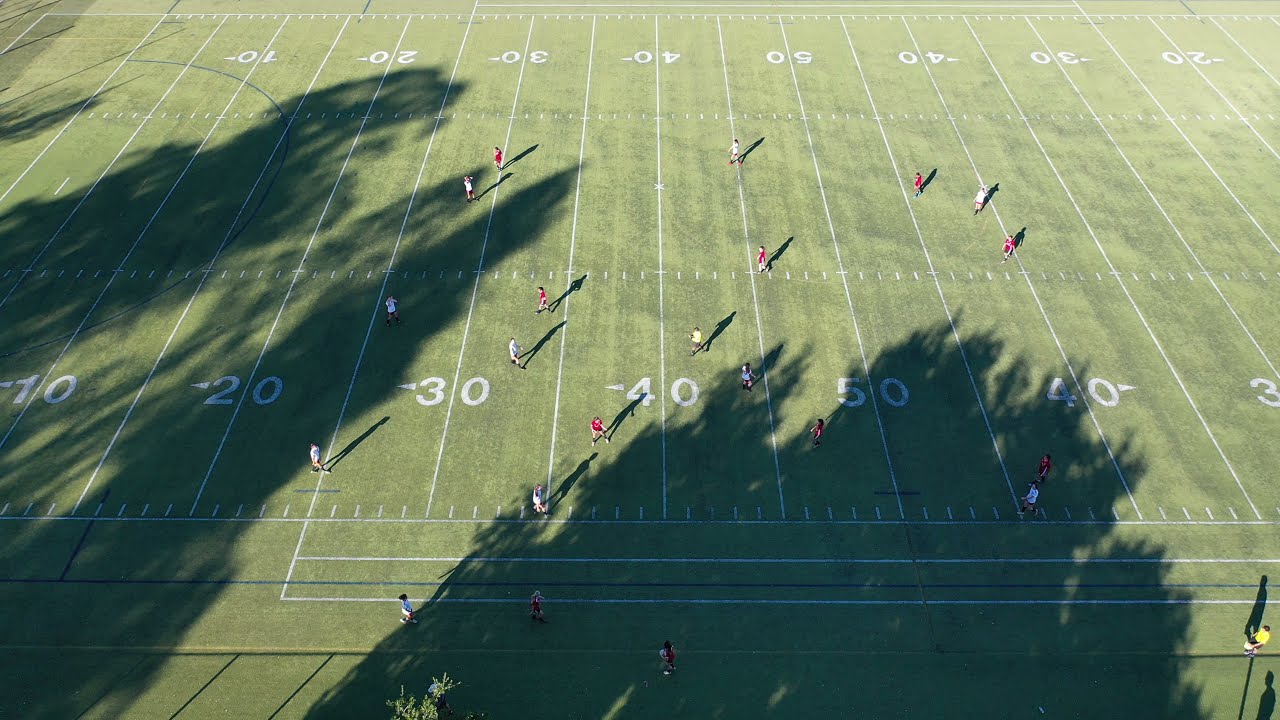This aerial photograph captures a football field from a significant altitude, allowing a comprehensive view of its layout and surroundings. The green grass field is marked with white yardage lines, showing the 10, 20, 30, 40, and 50-yard markers prominently as it stretches from left to right. At the top of the image, the end zone is visible, while the bottom part of the field cuts off just before the 30-yard line. There are numerous small figures on the field and the sidelines, appearing tiny and indistinguishable due to the high vantage point, with roughly half wearing red and the other half in lighter uniforms, which may be white. Long, dark shadows cast by large trees cover about a third of the field, suggesting the photo was taken either early in the morning or late in the afternoon. The significant height of the shot poses challenges in identifying specific details about the game, but it beautifully captures the scene's overall atmosphere and the interplay of sunlight and shadow.